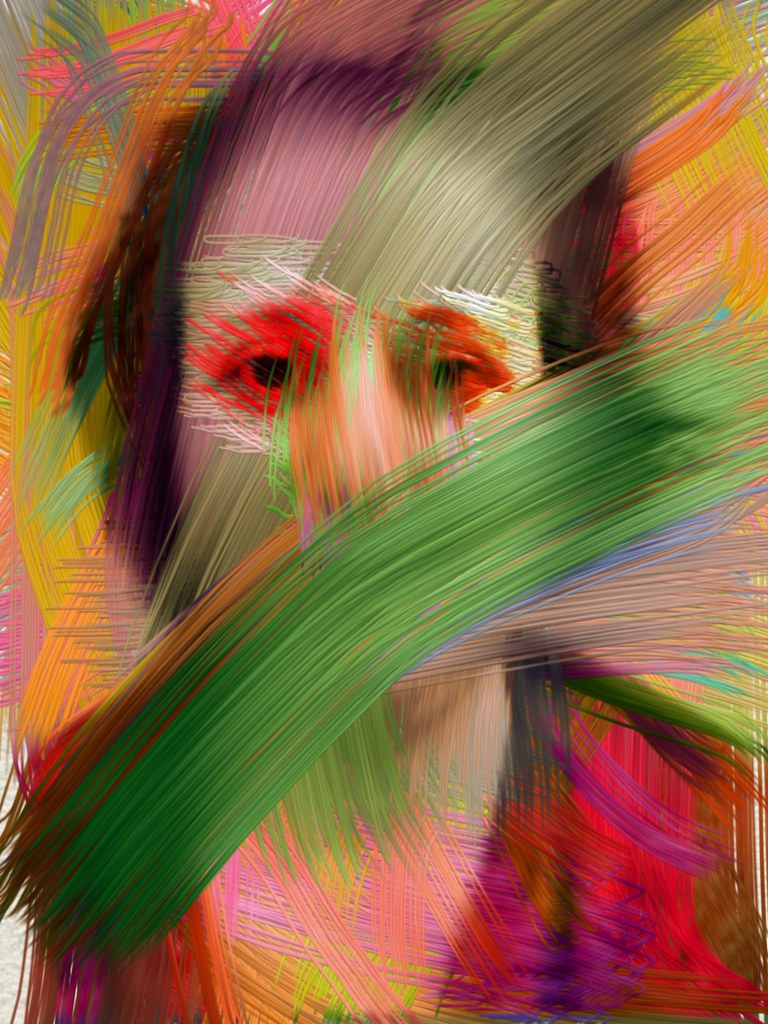The image depicts a striking digital illustration resembling an abstract self-portrait. The main focus is a close-up of a figure, possibly female or an older man, captured from the chest up, draped in a grey-colored nightgown or red shirt with a deep neckline. The subject's eyes, dark brown hair, and the side of the head are clearly discernible, although the nose and mouth are obscured by the painting's effects. The illustration is characterized by vibrant, smeared streaks of various colors, including neon hues of green, yellow, white, red, blue, orange, magenta, and pink. These colors blend seamlessly across the page, creating a chaotic yet harmonious backdrop that evokes the complex whirl of emotions, perhaps hinting at the artist’s mental landscape. The technique, likely created using a digital art program emulating oil paints, lends the figure a surreal, almost too-perfect appearance, where the interplay of colors both constructs and deconstructs the subject’s form, making them appear vividly real yet fundamentally abstract.